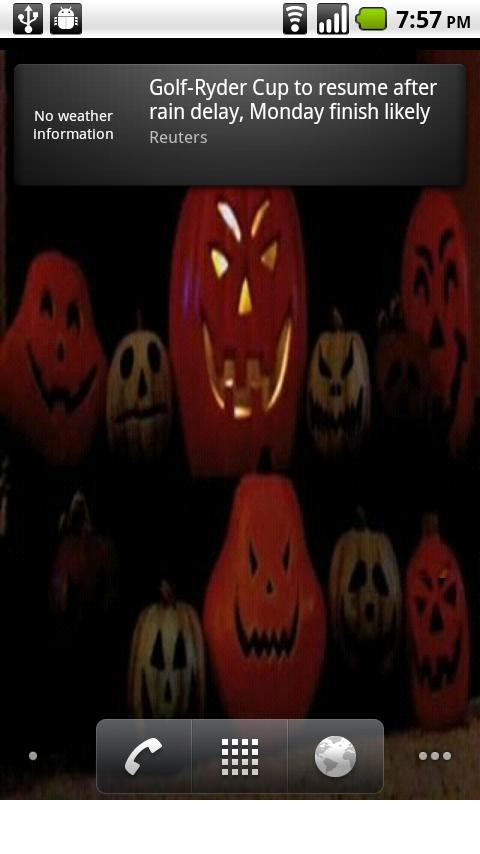A detailed screenshot of an Android phone is displayed, capturing various interface elements. At the very top of the screen, there is a silver notification bar. The bar includes several icons: a USB icon on the far left, followed by an icon resembling an alien or bug, and progressing to the right, there are icons for Wi-Fi, mobile signal strength, battery level, and the current time.

Beneath the notification bar, the desktop wallpaper is visible, featuring Halloween pumpkins with a very dark filter applied, giving the image a spooky ambiance. 

Overlaying the wallpaper, there is a prominent black pop-up rectangle at the top of the screen. The left side of this rectangle contains a message stating, "No weather information." Meanwhile, on the right side, the message reads, "Golf - Ryder Cup to resume after rain delay. Monday finish likely." The source of this alert is indicated as "Reuters."

At the bottom of the screenshot, three black navigation boxes are evident. The leftmost box includes a phone icon, the center box houses a keypad icon, and the box on the right features an earth icon, likely for internet browsing.